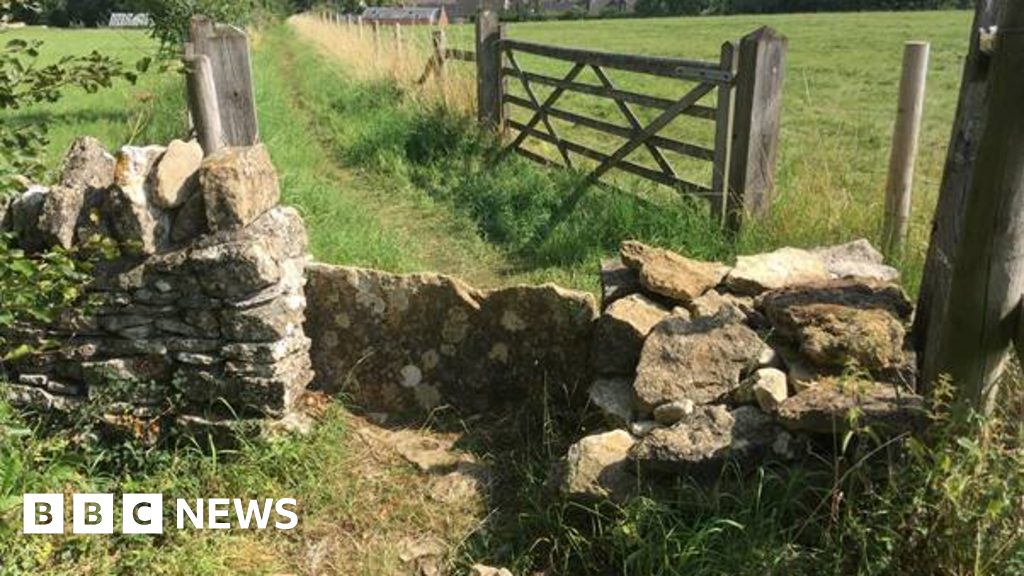The image, presumably a media shot or screenshot from BBC News, features their logo in white positioned in the bottom left corner. Dominating the scene is a lush field with green grass that appears to be over a foot tall. The central focus is on a stone wall composed of grey and brown rocks, situated in front of a wooden gated fence with posts on either side. This area creates a barrier and a sort of entrance outside the fence. The gate is distinctly open, adding to the inviting nature of the scene. Sparse dirt patches can be seen among the rocks and grass. Further in the background, under the clear daylight sky, a series of brick buildings are visible on the horizon to the right, complemented by other structures on the left. The sunlight illuminates the entire setting, enhancing the vibrant and clean look of this rustic landscape.